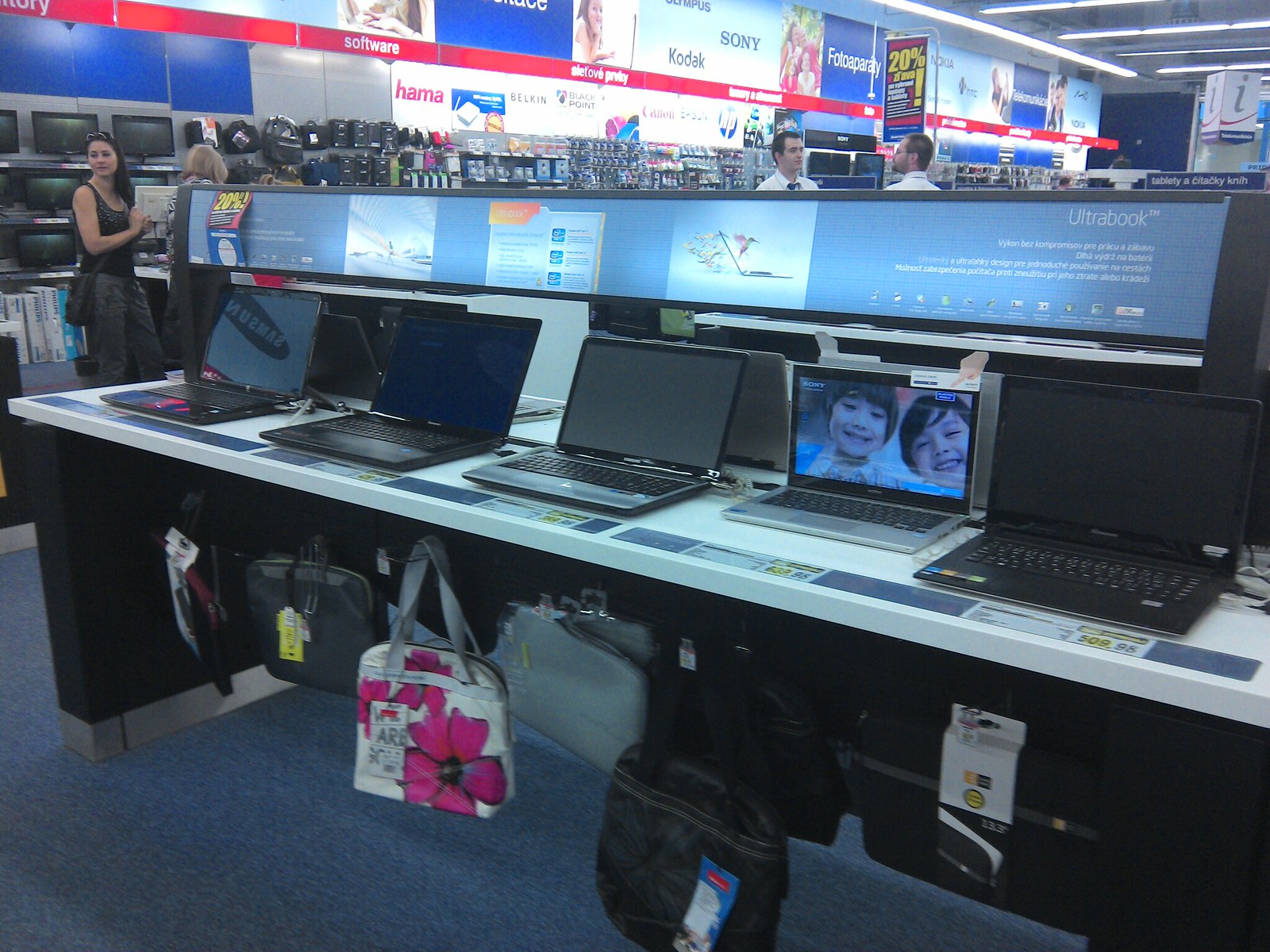This photo captures the interior of a bustling electronics store, likely similar to a Best Buy. At the forefront, there is a white counter showcasing five laptops, all in shades of grey and black, arranged in a neat row. One of these laptops is powered on, displaying an image of two children with dark hair, smiling at the camera. Blue price tags are affixed above each laptop, along a blue Ultrabook informational banner. Beneath the counter, various laptop bags in colors like black, brown, grey, and rose are visible, hanging from hooks.

Prominent advertisements decorate the store, including a red banner stating "software" and signs reading "Sony" and "Kodak photo party" in blue, alongside a "20% off" red sign. The background features further displays of monitors and other electronic accessories, underlining the store's extensive inventory.

In the scene, a woman in a grey top and pants stands to the left, while two salesmen dressed in white shirts and ties are positioned just behind the Ultrabook banner on the right. Their presence adds to the lively atmosphere of the store, filled with customers and electronic products on display.